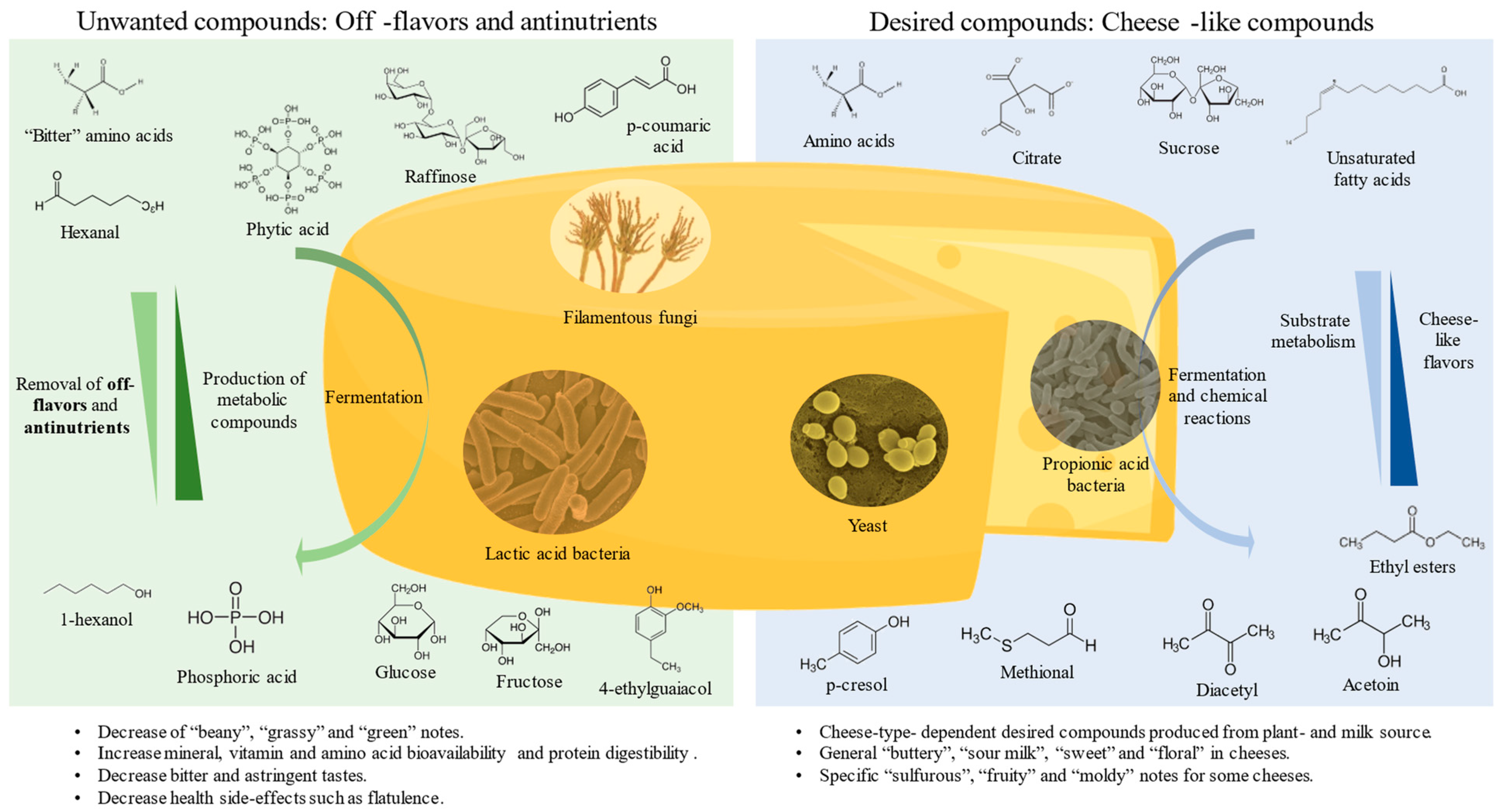This educational and scientific diagram features a detailed visual representation of cheese production and maturation, emphasizing the molecular structures and compounds involved. At the center, a large wheel of cheese with a wedge cut out highlights the various organisms and chemical processes crucial to cheese aging. 

On the left side, presented against a green background, are the unwanted compounds, off flavors, and anti-nutrients that negatively affect cheese quality. These elements can contribute to undesirable flavors such as grainy, bitter, beany, grassy, and green notes. 

On the right side, set against a blue background, are the desired compounds, or "cheese-like" compounds, which enhance the cheese’s flavor profile, contributing to buttery, milky, sweet, and floral characteristics.

The diagram intricately details the roles of different microorganisms like yeast, filamentous fungi, lactic acid bacteria, and propionic acid bacteria. It explains how these agents interact during the fermentation process, transforming initial ingredients into the wide array of complex flavors and textures found in matured cheese.